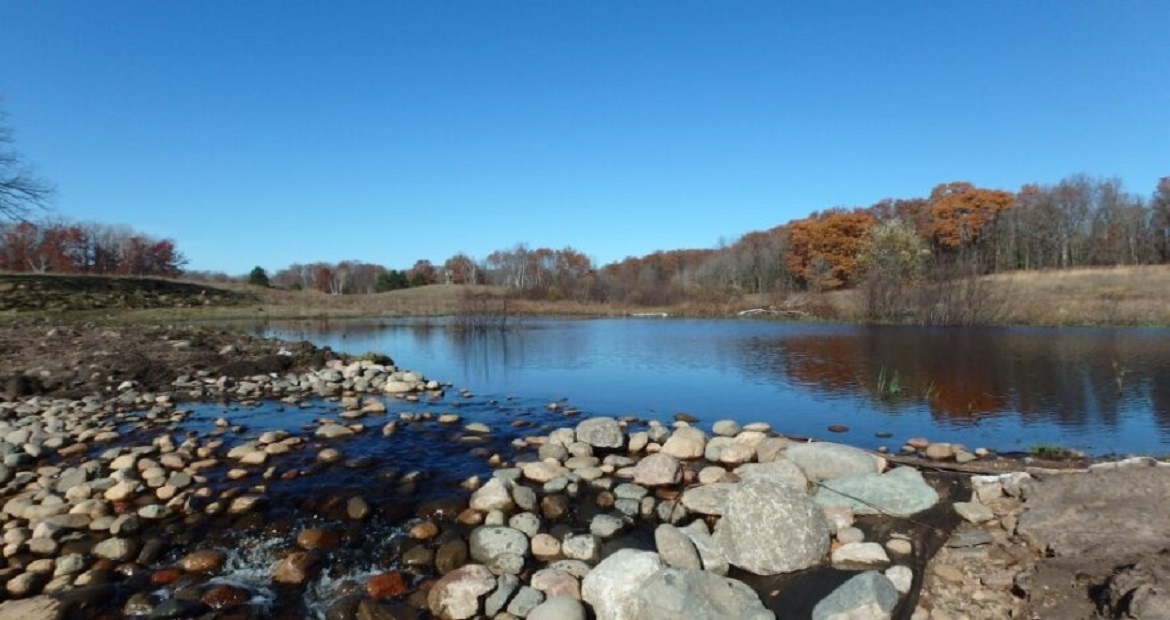This rectangular photograph captures a serene early spring pond, possibly nestled in New England. The top third of the image showcases a stunningly blue sky mirrored in the pond's tranquil waters. The middle section features the pond itself, reflecting the bare trees on a gently sloping hillside behind it. These trees, in their late autumn or early spring state, have dark brown leaves or are stripped bare, adding a rugged, seasonal charm to the scene. The bottom third emphasizes the large and small rocks lining the pond's edge, creating a natural outlet to a stream that likely begins right at this edge. The camera is positioned low, nearly at water level, emphasizing the splashing water as it overflows onto the rocks, which are interspersed with patches of grass and a stone wall visible on the left side of the frame. Despite the overgrown grass showing hints of a seasonal transition, the overall ambiance of the pond remains peaceful and inviting.